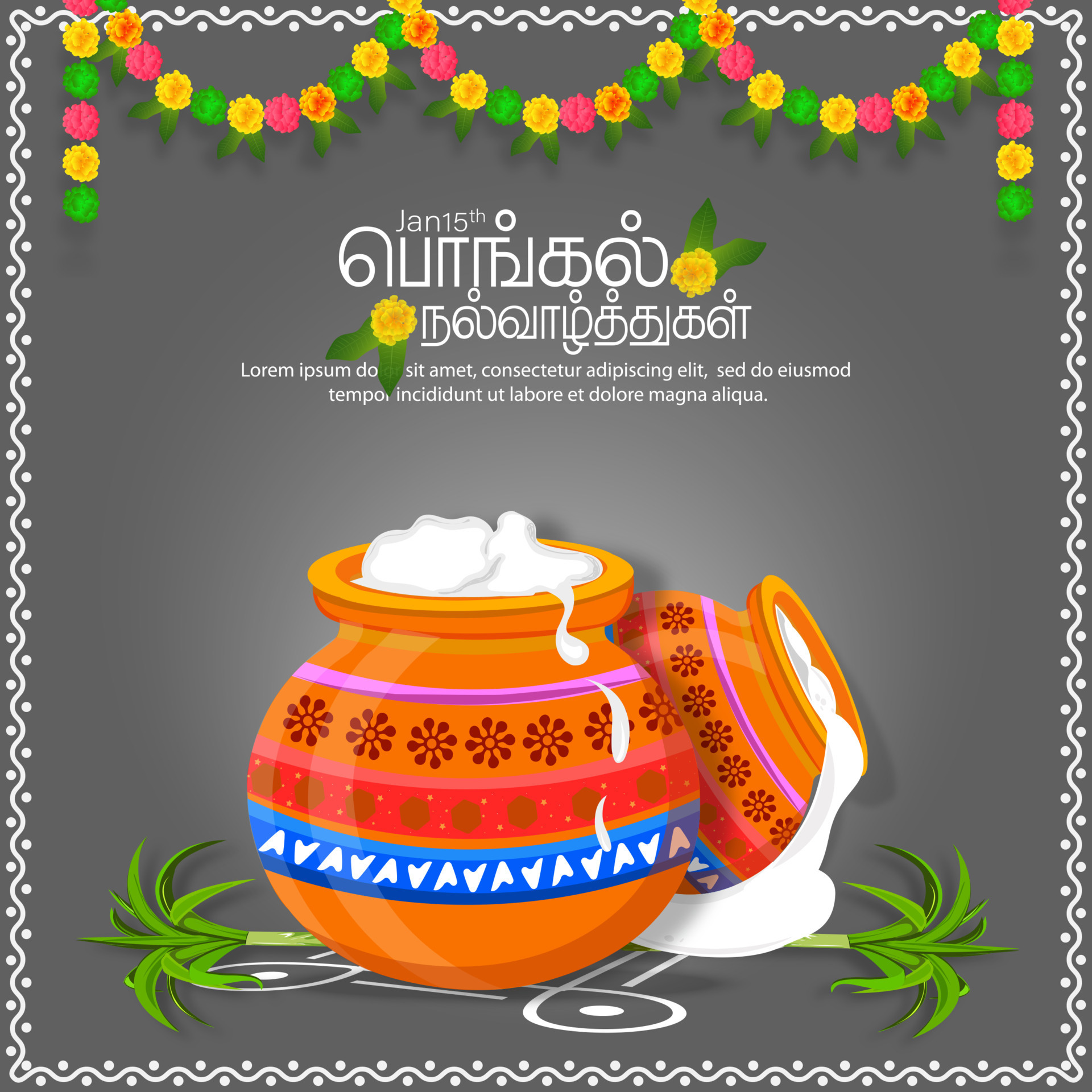This is a square digital graphic mock-up of a flyer with a gray background, intricately detailed with an Indian-inspired theme. The flyer features a top banner adorned with alternating yellow, pink, green, and orange flower garlands, symbolic of Indian tradition. The border of the flyer is decorated with a wavy white line interspersed with small circles. At the top, the date "January 15th" is prominently displayed, using a large, swirly white font alongside some non-English text, possibly in an Indian language. The main body showcases an illustration of two orange, ceramic-like jars. One jar is upright with a thick, white, creamy substance overflowing, while the other jar is tilted, spilling the same substance. The jars are intricately decorated with a pink border, dark red and gold floral patterns, and a blue stripe featuring repeated letters "A" and "B." Additionally, small green stems and a flower accent are depicted near the jars, contributing to the overall aesthetic. The text below the illustration appears to be placeholder text in a lorem ipsum font, indicating that the flyer is still a work in progress.